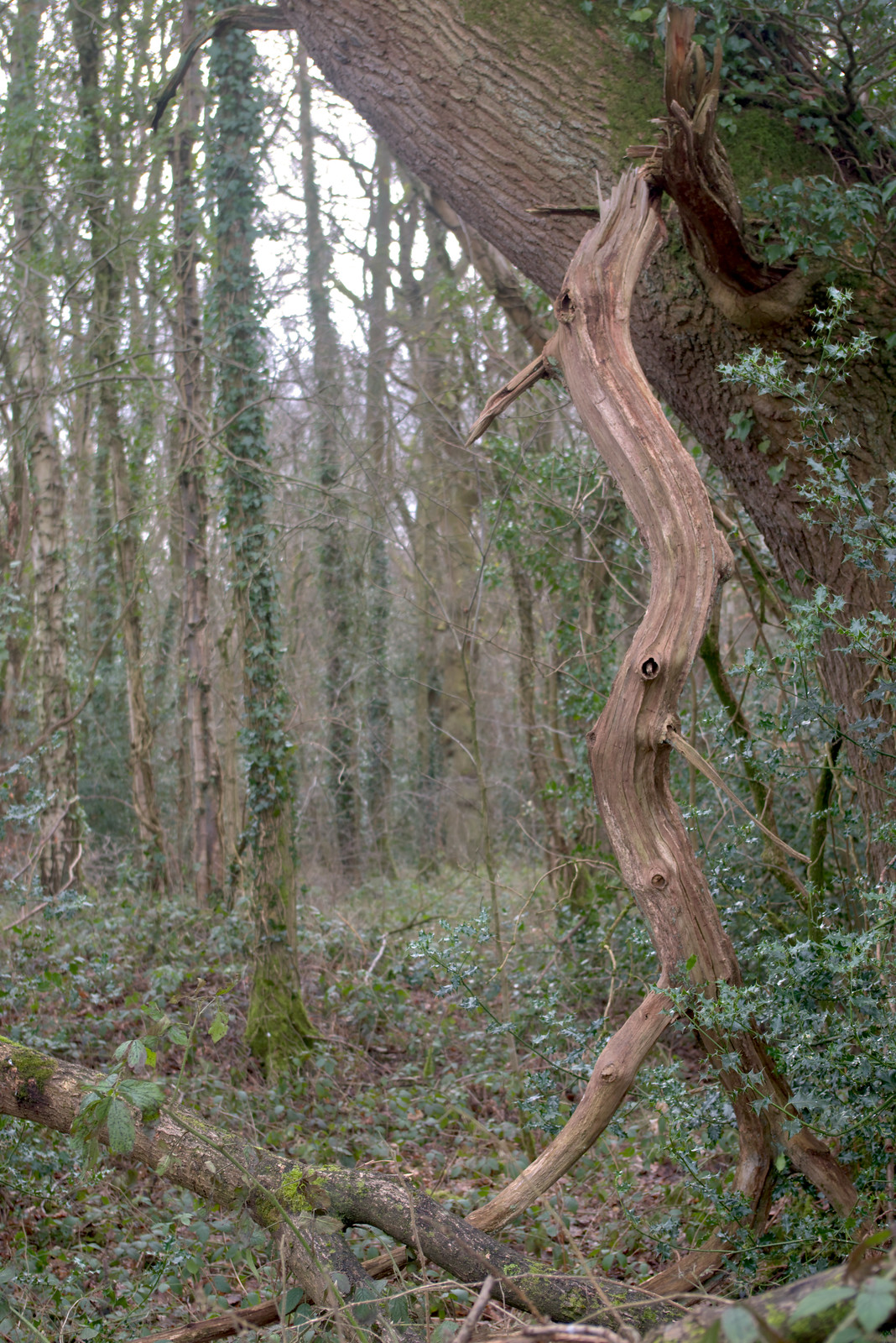The photograph depicts a serene forest scene bathed in daytime light, with a light gray sky peeking through a canopy of varied tree branches. The foreground features several dead branches, barren of leaves, with one standing vertically, barely clinging to a tree trunk above it. The forest is sprinkled with thin trees, some adorned with green leaves, others with bare branches, and many enveloped by vines and moss. Amidst the trees, one distinctive figure-like tree stands out, resembling a walking creature with a pointy nose, an eye-like hole, and branches mimicking limbs. The ground is a tapestry of small ferns, grasses, and vines, punctuated by patches of dirt. The scene is lush yet not densely populated, giving it an airy, mystical atmosphere.